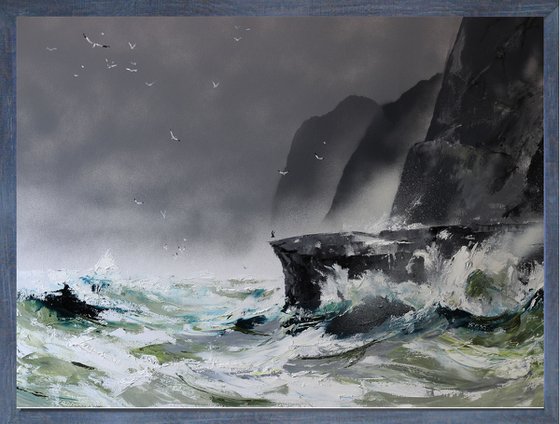This highly detailed watercolor painting, encased in a blue wooden frame, captures the wild beauty of a rough ocean scene. Dominated by shades of gray, white, and green, the crashing waves send sprays of foam against the cliffs on the right side of the image. At the edge of the foremost cliff, a small humanoid figure stands, steadfast against the turbulent water. Seagulls, some with black-tipped wings, populate the dark gray and light gray skies, adding life above the chaos. The sky is thick with gray clouds blending into the misty ocean air, while hints of blue and dark blue ripple through the waves and create a sense of depth. The cliffs in the background rise tall and imposing, enveloped in a smoky haze that merges with the distant clouds.